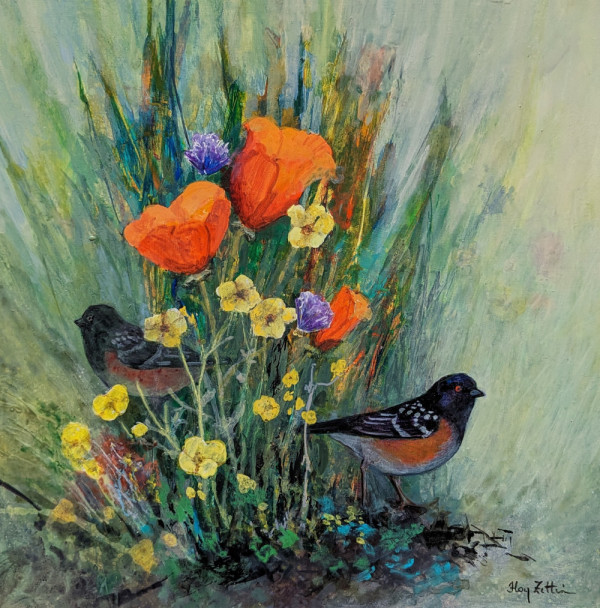The painting showcases a vibrant and intricate cluster of various species of flowers sprouting from a base of black soil. The diverse array of flowers, displayed in rich hues of yellow, purple, and orange, adds depth and texture to the composition. Perched on the ground among these blossoming flowers are two identical birds. Each bird is exquisitely detailed with brown legs, white stomachs adorned with orange spots, black wings with white accents, black heads with striking orange eyes, and small, conical black beaks. The background is a luscious green that accentuates the colorful foreground.

Additionally, the painting features a signature and an inscription in elegant calligraphy at the bottom right corner, indicative of the artist's personal touch. The entire piece is framed, without any accompanying text, allowing the vivid colors and meticulous details to captivate the viewer. The major colors in this artwork include various shades of orange, yellow, lilac, green, blue, black, and white, seamlessly blended to create a harmonious and visually stimulating masterpiece.